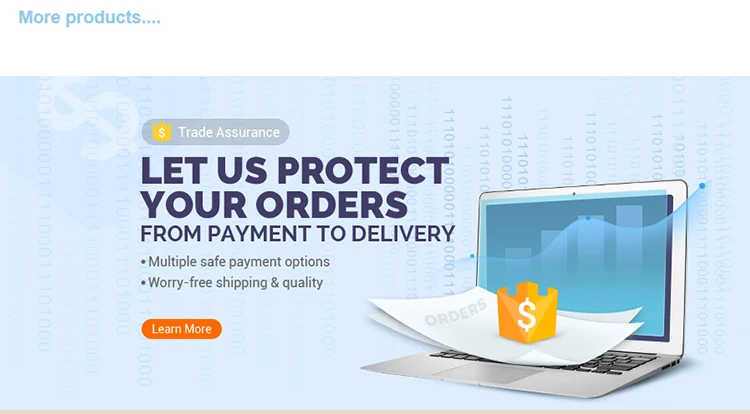The image depicts a section of a website's landing page. In the top left corner, the text "More Products...." is displayed in a powdery sky-blue color. Below this text, there is a white gap approximately an inch thick. Beneath this white space, a sky-blue box occupies the section featuring faint white dollar signs and vertically running binary code in light gray, reminiscent of scenes from the Matrix movies.

At the center top of this box, there is a gray bubble containing a gold and white dollar sign icon, accompanied by the text "Trade Assurance." Below this, the subtitle reads, "Let us protect your orders from payment to delivery." The section also highlights two key benefits: "Multiple safe payment options" and "Worry-free shipping and quality."

Towards the bottom, an orange and white bubble with the text "Learn More" invites further engagement. On the right side of the image, there is a laptop with white papers labeled "Orders." The gold dollar sign icon appears again on top of these papers and the laptop, reinforcing the theme of secure transactions.